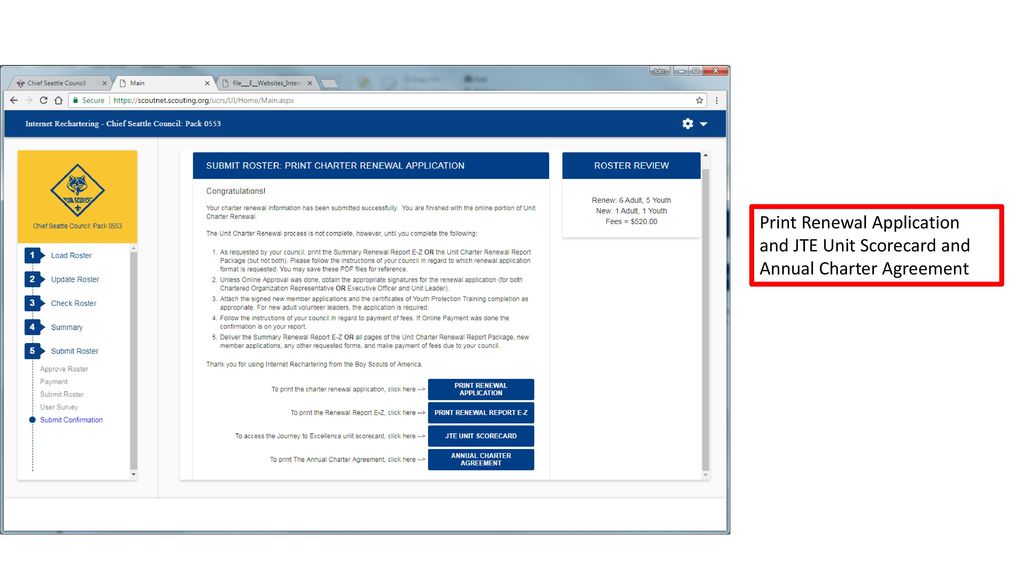The image depicts a computer interface brimming with various navigational and operational elements. At the top, there are several gray tabs with an "X" on each to close them. Directly below, a long white search bar is prominently displayed, accompanied by a green lock icon and the word "Secure" to its left, suggesting a secure connection.

Following this is a horizontal blue bar extending across the screen, featuring a settings wheel icon positioned on the far right. Below the blue bar on the left side, there is a distinctive yellow square containing a diamond shape, which encapsulates the image of a fox. Beneath this graphic are four blue text options: "Load," "Update," "Check," and "Submit."

To the right side of the interface, under a blue background, there is a section titled "Submit Roster, Print Charter Renewal Application." Adjacent to this title is another indicating "Roster Review," accompanied by a list of five bullet points, each followed by a few sentences in small black text.

Towards the bottom of the interface, there are four blue boxes, each with white text inside, although the specific text within these boxes is not detailed. On the far right, a red square stands out, containing black text that reads "Print Renewal Application, JTE Unit Scorecard, and Annual Charter Agreement." 

The interface layout is a mix of vibrant colors and functional elements designed to facilitate user interaction and navigation.